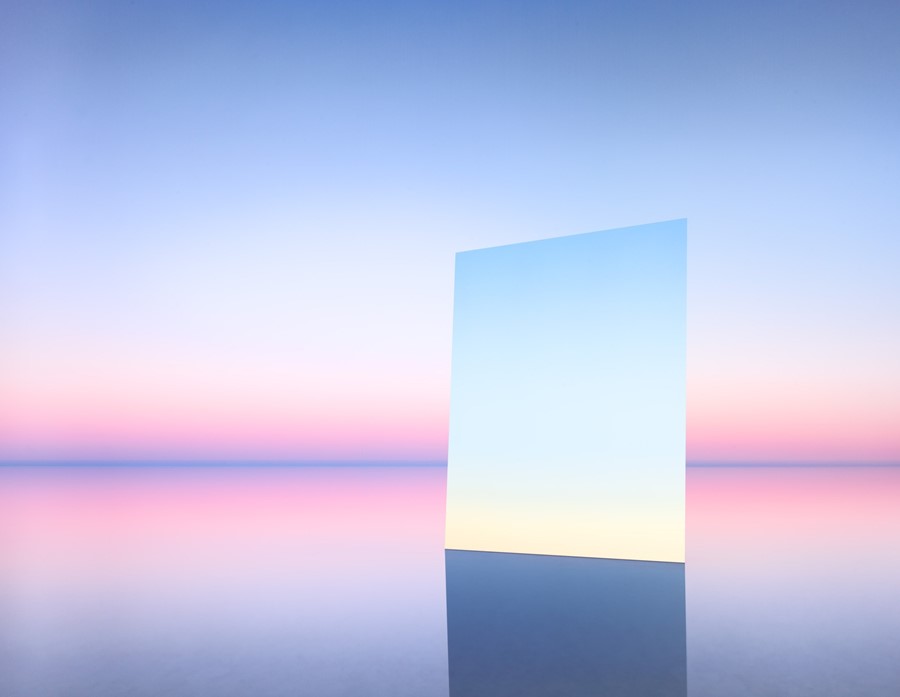The image appears to be a digitally created abstract space composed of a single rectangular surface displayed at an angle, giving it an uneven look, as if it were a flat 2D plane without a 3D effect. The rectangle features a gradient coloring that starts with a light blue at the top and fades into a nearly white or pale yellow hue at the bottom. Below this shape, there's a distinct shadow in dark blue or gray, emphasizing the light source and adding depth. 

The background of the image is characterized by a gradient that starts with dark blue at the very top, fades into light blue, transitions to light pink, and deepens to dark pink toward the bottom, creating a visually pleasing effect reminiscent of a sunset. About a third of the way up from the bottom, a thin dark blue line runs horizontally across the image, mimicking a horizon line and helping to define the space. This line also enhances the illusion of a blue floor and wall extending from the corner.

Overall, the central element, which looks like a square or a slightly distorted cube, stands out against the vibrant, colorful background, offering a striking contrast and visual interest.